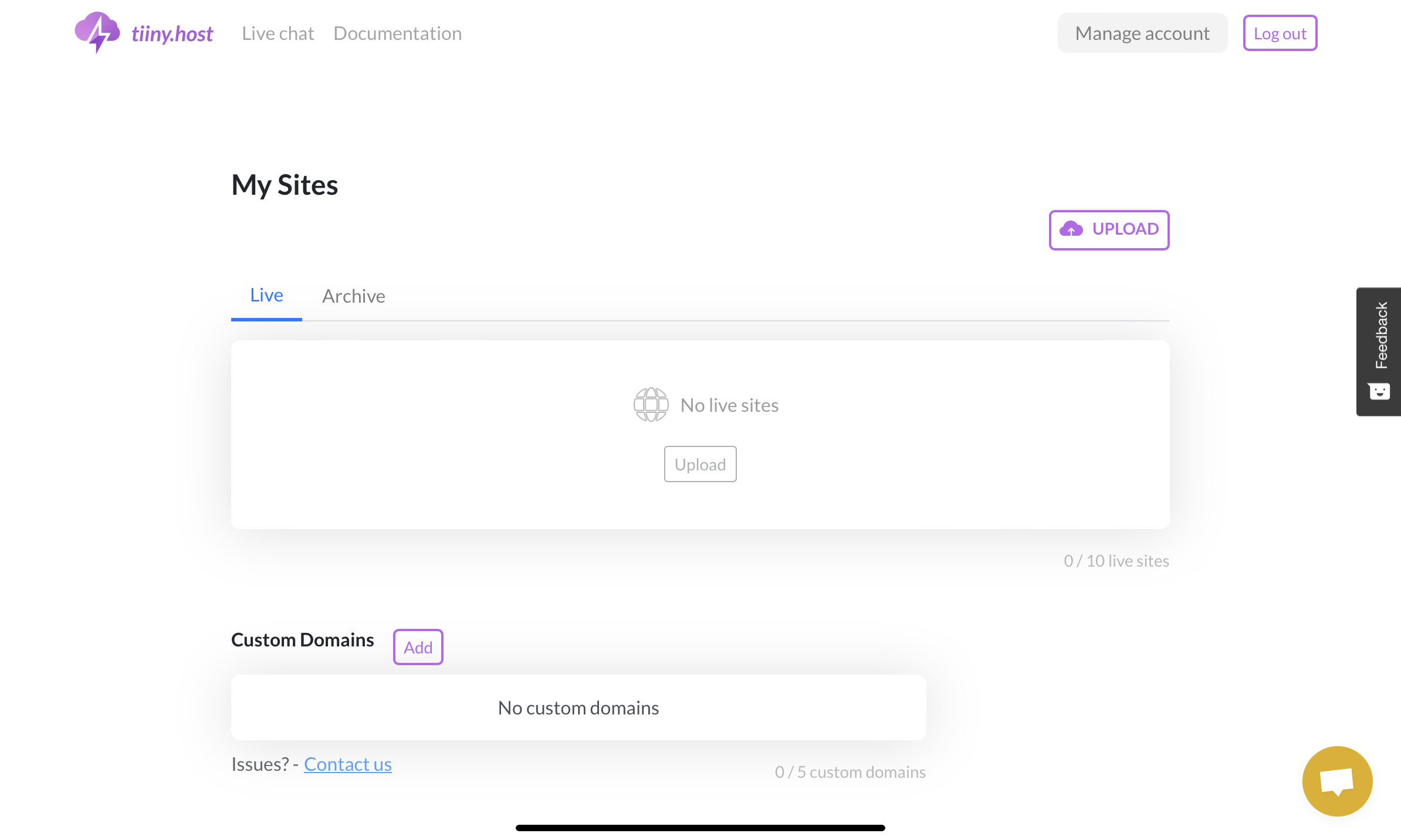The image showcases a webpage from tiny.host, spelled as T-I-I-N-Y dot host. The logo, situated in the top-left corner, features a purple cloud with a lightning bolt striking down through its center. To the right of the logo, there are two tabs: "Live Chat" and "Documentation." Further right, a gray "Manage Account" button is followed by a purple-circled "Logout" button.

In the main body of the page, a section titled "My Sites" appears on the left. Directly below this section, there are two tabs: the current tab "Live" and an adjacent "Archive" tab. Next to these tabs is a purple "Upload" button. Beneath this, an icon of a globe indicates no live sites are available, accompanied by another "Upload" button.

Continuing downwards, there's a status indicator showing "0/10 Live Sites." Below it, there's a "Custom Domains" section with an "Add" button, also in purple. The section notes "No Custom Domains" and displays a status of "0/5 Custom Domains." At the lower right, a chat bot icon is present alongside a black "Feedback" button.